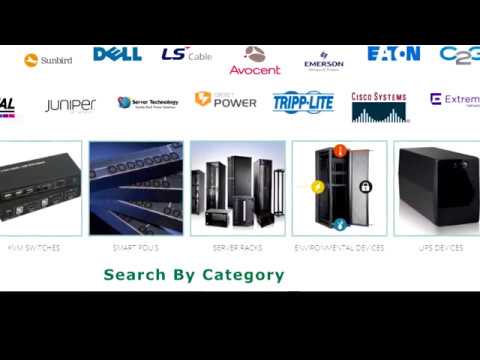The image showcases a comprehensive array of company logos arranged in a grid-like fashion at the top. Notable companies featured include Sunbird, Dell, LS Cable, Avocent, Emerson, Eaton, Juniper, Triplight, Cisco Systems, and others, signifying a diverse range of industry leaders. Directly below the logos, five square images display various computing components, though the accompanying text below each image is blurry and low quality, rendered in a light gray font that is difficult to decipher. At the bottom of the image, near the center, a message in green text reads "Search by Category." The entire composition is set against a white background, framed with black bars at the top and bottom, creating a balanced and organized layout.